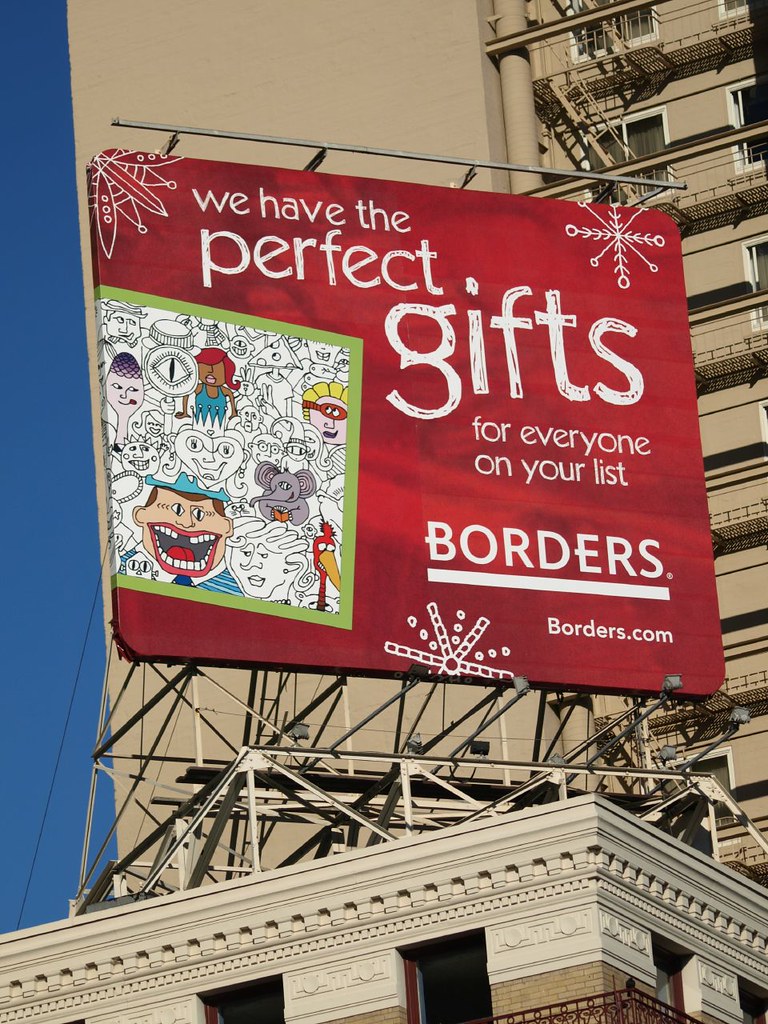The photograph depicts a prominent billboard mounted atop a stone building. The building occupies the bottom 10-20% of the image and features a decorative whip-like design below its flat roof. The stone has a light brown hue. Rising above it in the background is a tall apartment complex characterized by grayish beige taupe brick and visible fire escapes on the right side, with metal ladders and flooring on each level.

The billboard, roughly square with rounded corners, is the central focus. It has a predominantly red background adorned with white text and stenciled snowflake designs. The text reads, "We have the perfect gifts for everyone on your list," in handwriting-styled lettering spread across the billboard's center. The lower right corner features the Borders bookstore logo in white block letters, underlined by a horizontal white line, followed by "Borders.com".

On the left side of the billboard is a green square containing abstract cartoon-style faces, resembling a page from a coloring book, with some faces uncolored. The overall scene is set against a clear blue sky, emphasizing the festive holiday advertisement by Borders.